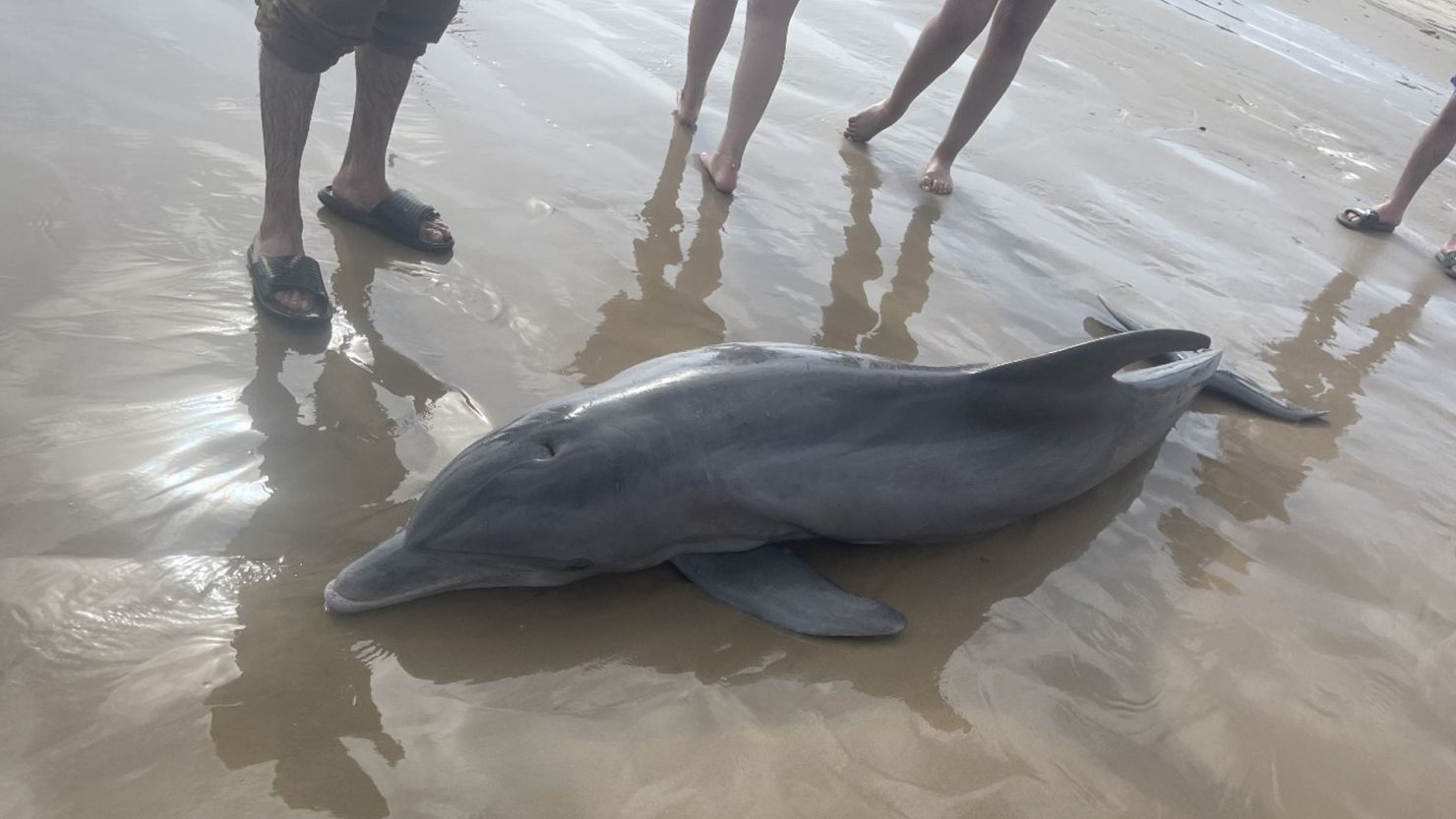The photograph captures a somber scene of a bottlenose dolphin washed up on a shore, lying on its belly in the wet, dark beige sand with its tail to the right and nose to the left. The scene is set near the water's edge, where the sand appears wet from recent waves, but there is drier sand further behind. Surrounding the stranded dolphin are four people, visible only from the knees down. On the top left corner stands a person with brown pants rolled up and wearing leather sandals. Among the group, two individuals are barefoot and appear to have feminine feet, while another person on the right side is in flip-flops. The sun casts its light on the tableau, highlighting the glistening gray body of the dolphin as the onlookers stand, seemingly contemplating or perhaps deciding on how to respond to the dolphin’s plight.